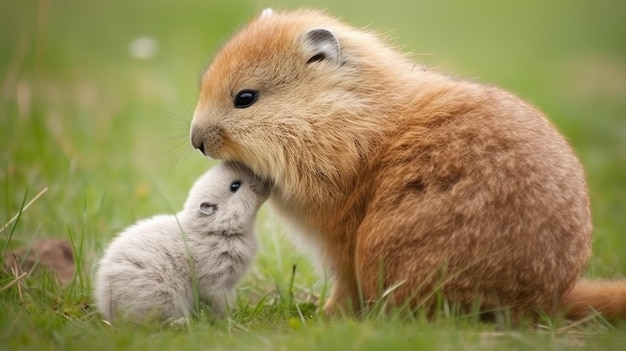The photograph captures a heartwarming scene of two cute, furry rodents, possibly hamsters or some type of small rodent, nestled together in a grassy area. The larger rodent has light brown, almost golden fur with short, rounded ears and striking black eyes, and features a long tail partially visible in the background. The smaller rodent, positioned endearingly under the chin of the larger one as if nuzzling, is a creamy or almost white color with similar dark eyes and slightly darker grayish ears. The grassy terrain they are situated in appears lush and natural, akin to a park setting, with the focus centered sharply on the affectionate pair, making the surrounding grass appear blurred. Additionally, there seems to be a hint of another rodent or object to the left, though it remains indistinct. The overall effect of the composition highlights the adorable interaction between the two animals, evoking a sense of tenderness and familial bonding.